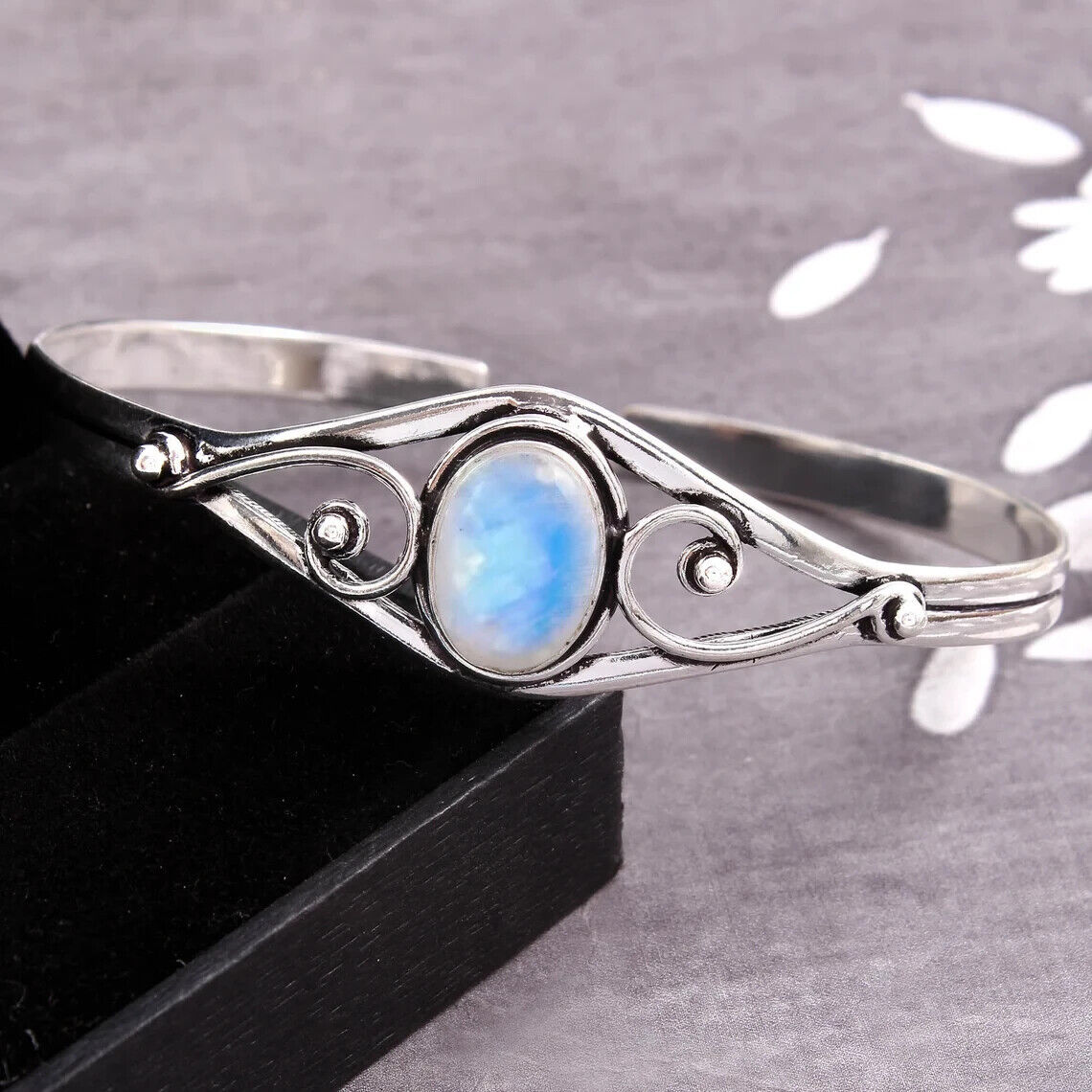The image showcases a detailed close-up of a silver bracelet, elegantly resting on the edge of a black wooden board positioned to the left side against a gray background. The bracelet features a larger central area with an upward and downward curve, prominently displaying an oval-shaped, light blue gemstone that shimmers like moonstone. Flanking the gemstone are intricately designed, vine-shaped silver metal embellishments, each ending with a small, sparkling crystal. Subtle elements, such as bits of white and what appears to be a velvet-lined black case, enhance the luxurious feel of the composition. The backdrop includes a piece of silver fabric, contributing to the overall sophisticated and muted color palette of the photograph.